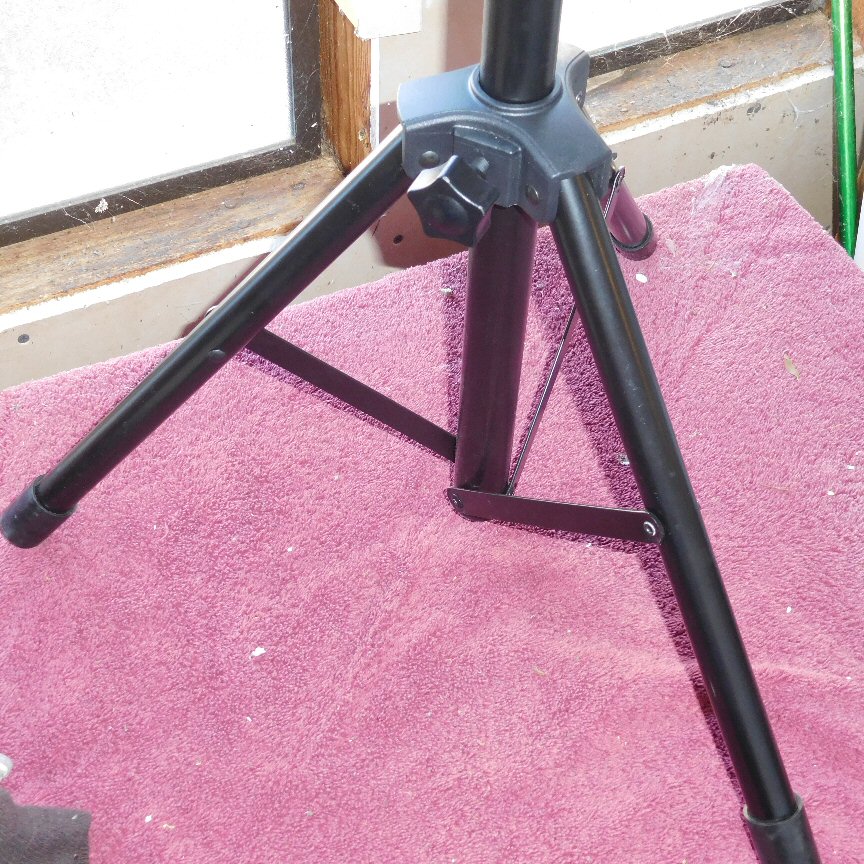The image showcases a black metal tripod with three pronged legs, each extending in different directions. The tripod is positioned on a pink or purple carpet within a room. The surrounding floor appears wooden, and the wall is white drywall with an aged wooden window frame. Cobwebs adorn the window frame, emphasizing its old and somewhat dirty condition. Bright white light streams through the window, making it impossible to discern the scene outside, likely due to sunlight reflecting off the glass. A green hose is visible near the base of the tripod, appearing to lead out of the window. The tripod's central pole rises up but its top is out of the frame, leaving it unclear whether it supports a camera, scope, or another device. Additionally, the third leg of the tripod seems slightly raised, causing the structure to lean a bit to the right.